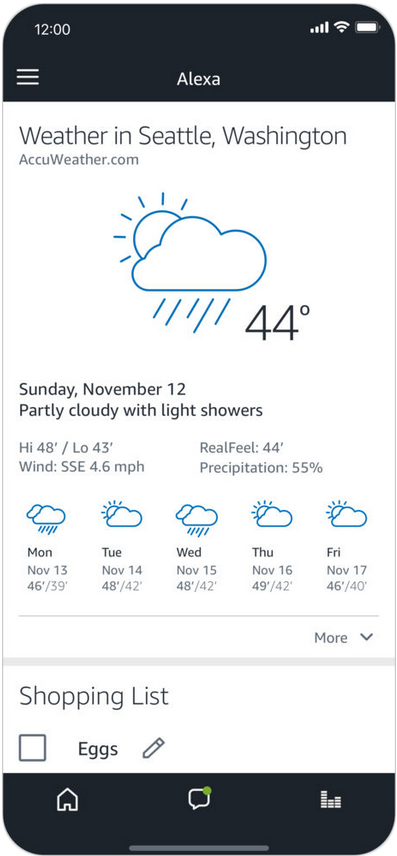The screenshot displays a weather report for Seattle, Washington, provided by AccuWeather.com. At the top-center, the word "Alexa" is prominently featured, indicating that this weather report might have been accessed via an Alexa-enabled device. Below this, the report clearly indicates the current weather conditions in Seattle. 

The temperature is 44 degrees Fahrenheit, accompanied by an icon depicting a cloudy sky with a partial sun and light rain. This signifies partly cloudy conditions with light showers. The report specifies additional details including:

- Date: Sunday, November 12
- Expected weather: Partly cloudy with light showers
- Temperature specifics: High of 48 degrees, low of 43 degrees
- RealFeel® temperature: 44 degrees
- Wind: SSE 4.6 mph
- Precipitation chance: 55%

Additionally, the bottom portion of the screenshot includes weather predictions for the upcoming weekdays, from Monday through Friday of the same week, although specific details for these days are not provided in the caption.

This detailed weather report helps Seattle residents prepare for their immediate and upcoming weather conditions.